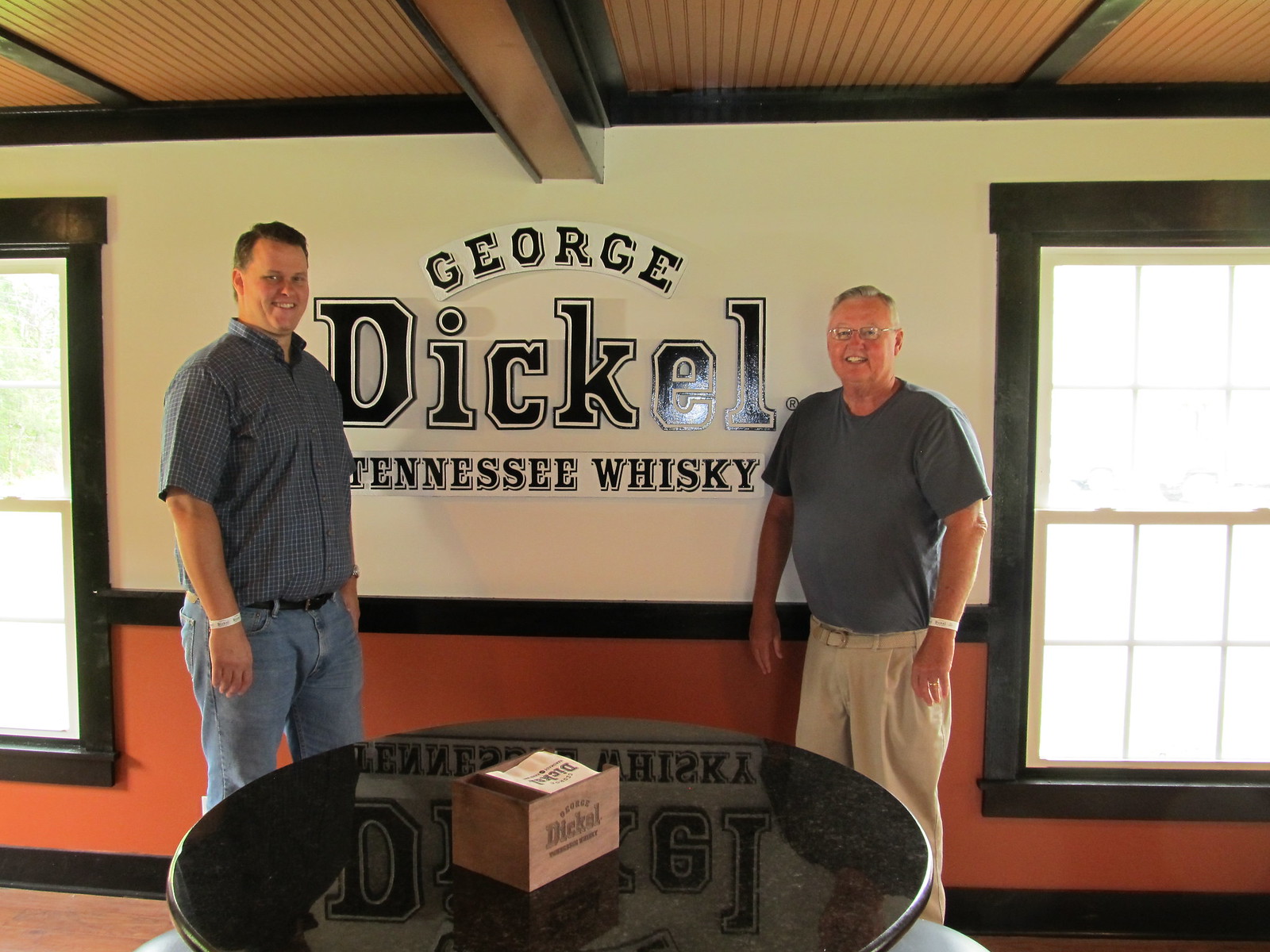This indoor photograph, potentially taken inside a distillery or bar, captures two men standing side by side in front of a wall with brown text that reads "George Dickel, Tennessee Whiskey." The wall behind them is off-white with some brown wainscoting and features two windows that allow sunlight to stream into the room, illuminating the scene. 

To the left is a younger man, likely in his 30s or 40s, who is moderately overweight. He is dressed in a white, short-sleeved, collared shirt, blue jeans, and a wristband, smiling directly at the camera. To the right stands an older man, probably in his 60s, also slightly overweight. He wears glasses, a gray or green t-shirt, khaki pants with a webbed belt, and a name band identical to the younger man's. He too is smiling warmly.

Between the men stands a dark circular table, possibly black marble, with a wooden box on top. The box reads "George Dickel," reinforcing the distillery branding. This posed picture, with detailed elements and the men’s casual attire, likely serves to advertise or celebrate the distillery, capturing a warm and welcoming scene.